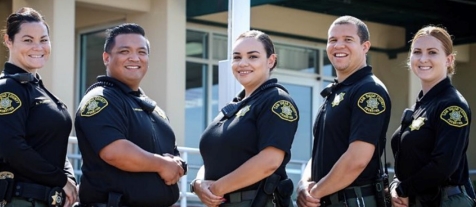This photograph features five individuals clad in matching black uniforms, indicative of a security force or police group, standing outside in daylight in front of a building. The uniforms are adorned with a distinctive patch on their shoulders, showcasing a six-pointed star, though the precise logo details are indistinguishable. The composition captures three females and two males, arranged with the females at the first, third, and fifth positions and the males at the second and fourth. The group exhibits a split stance; the three individuals on the right side are facing the two on the left, yet all five are looking directly at the camera. Notably, the central three individuals are in short-sleeved uniforms, while the females on the outer ends wear long-sleeved versions, adding a subtle variation to their coordinated attire. The bright sunshine highlights the professionalism and readiness of the group.